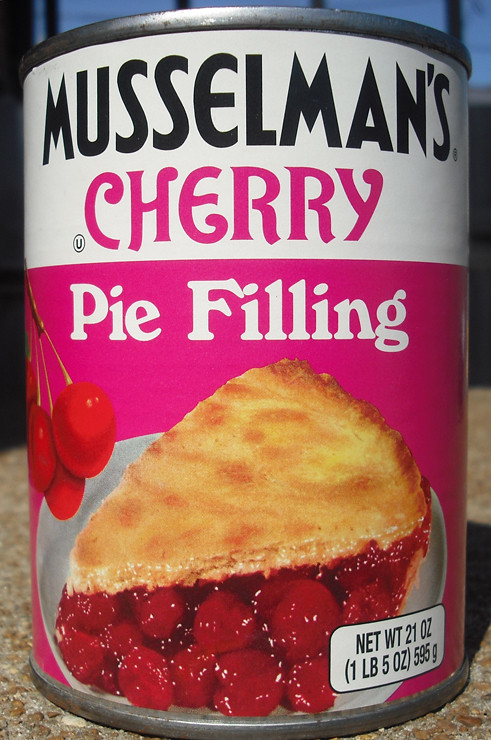This image features a close-up of a can of Musselman's Cherry Pie Filling, prominently displayed on a table. The label is divided into two main sections: the upper part has a white background with the brand name "Musselman's" written in a combination of navy blue, cherry, and pink hues. The lower section of the label is pink, adorned with vibrant cherries, the text "Pie Filling" displayed in white, and an appetizing image of a slice of cherry pie on a white plate. The can's label also indicates the net weight as 21 ounces, or 1 pound 5 ounces, equivalent to 595 grams. In the background, partially visible is a window, suggesting that it is dusk or nighttime outside.